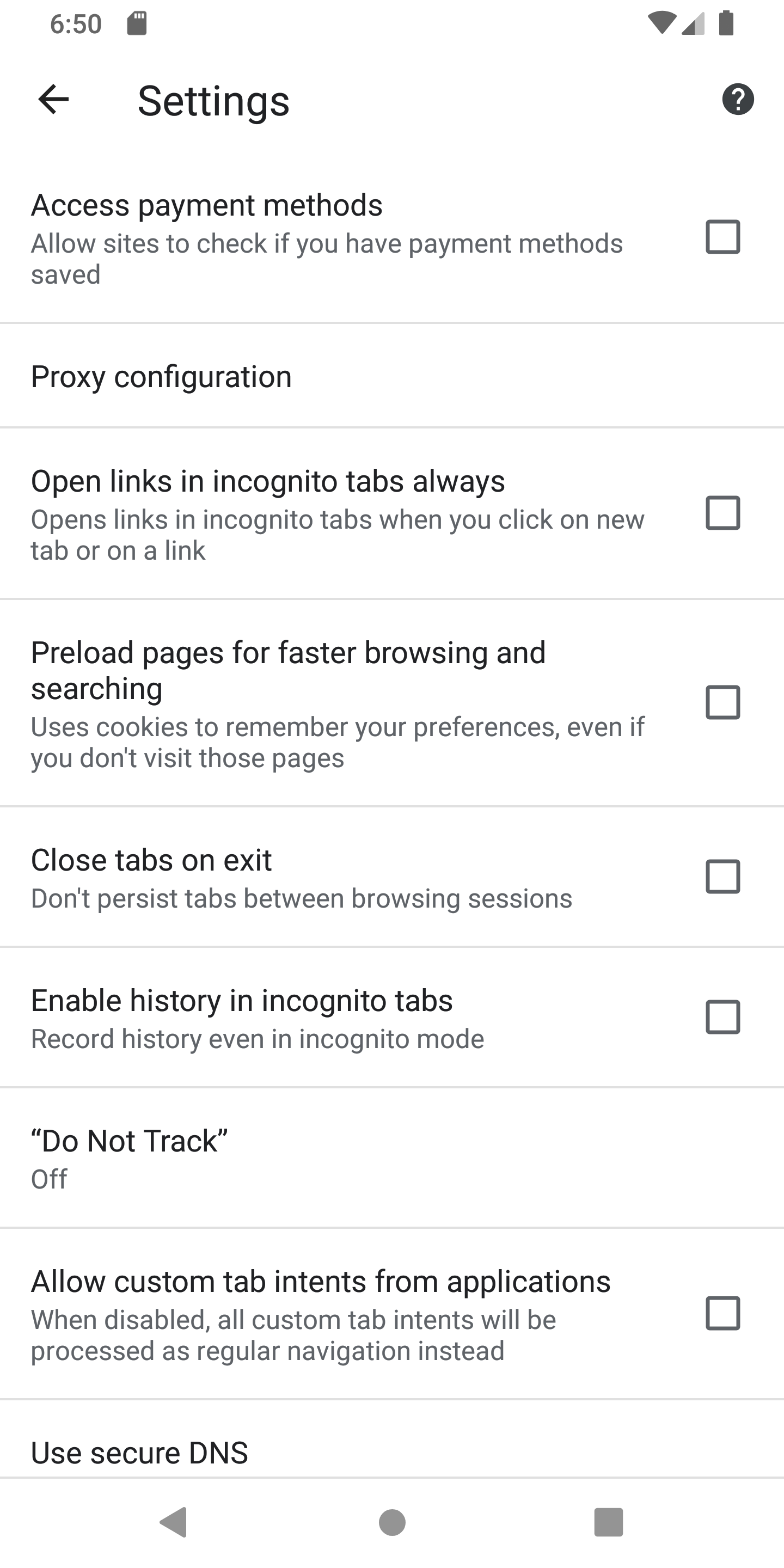This image showcases the settings page of a browser on a smartphone. At the top of the screen, standard smartphone icons are visible, including indicators for battery life, Wi-Fi signal, and the time, which is 6:50. Directly below these icons, a left-facing arrow is situated on the left side of the screen, adjacent to the word "Settings."

The main section of the page contains a series of options, each separated by a gray line, with clickable checkboxes on the right side for some of the choices:

1. "Access payment methods" – with an accompanying explanation.
2. "Proxy configuration" – without a checkbox.
3. "Open links in incognito tabs always."
4. "Preload pages for faster browsing and searching."
5. "Close tabs on exit."
6. "Enable history in incognito tabs."
7. "Do not track" – listed as off and without a checked box.
8. "Allow custom tab intents from applications."

Additionally, there is an option labeled "Use secure DNS," which also does not have a checkbox next to it.

At the bottom of the screen, there are three navigation icons in gray: a left-facing triangle, a circle, and a square.